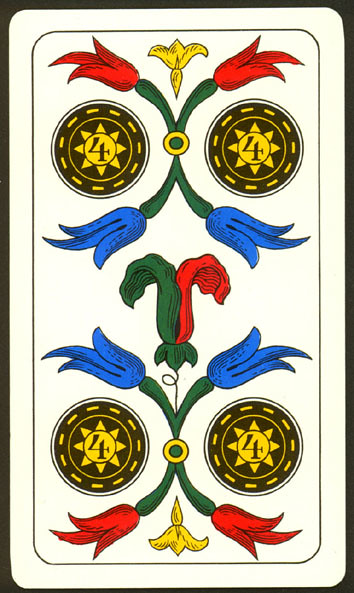Here we have a detailed illustration of a tarot card. The card maintains the traditional rectangular shape with neatly defined corners. The central focus of the card is a smaller rectangle that holds intricate designs. Inside this rectangle, there are four coins arranged symmetrically, two at the top and two at the bottom.

Each coin features a street-like design on a black background with yellow markings that emulate roads. In the center of each coin is a smaller circle containing an image of the Sun and the number four. The number is prominently placed within the Sun, adding emphasis to the count.

The center of the card showcases a distinctive rose that is half green and half red, symbolizing a unique blend of elements. Surrounding this central rose, the card displays ornate floral patterns reminiscent of traditional playing cards. These patterns consist of V-shaped arrangements of blue flowers pointing upwards and red flowers pointing downwards. Nestled between the red flowers, there is a yellow flower, further enhancing the intricate design.

Overall, the elaborate details and symmetrical arrangements contribute to the card’s ornate and captivating appearance, drawing the observer into its rich symbolism.